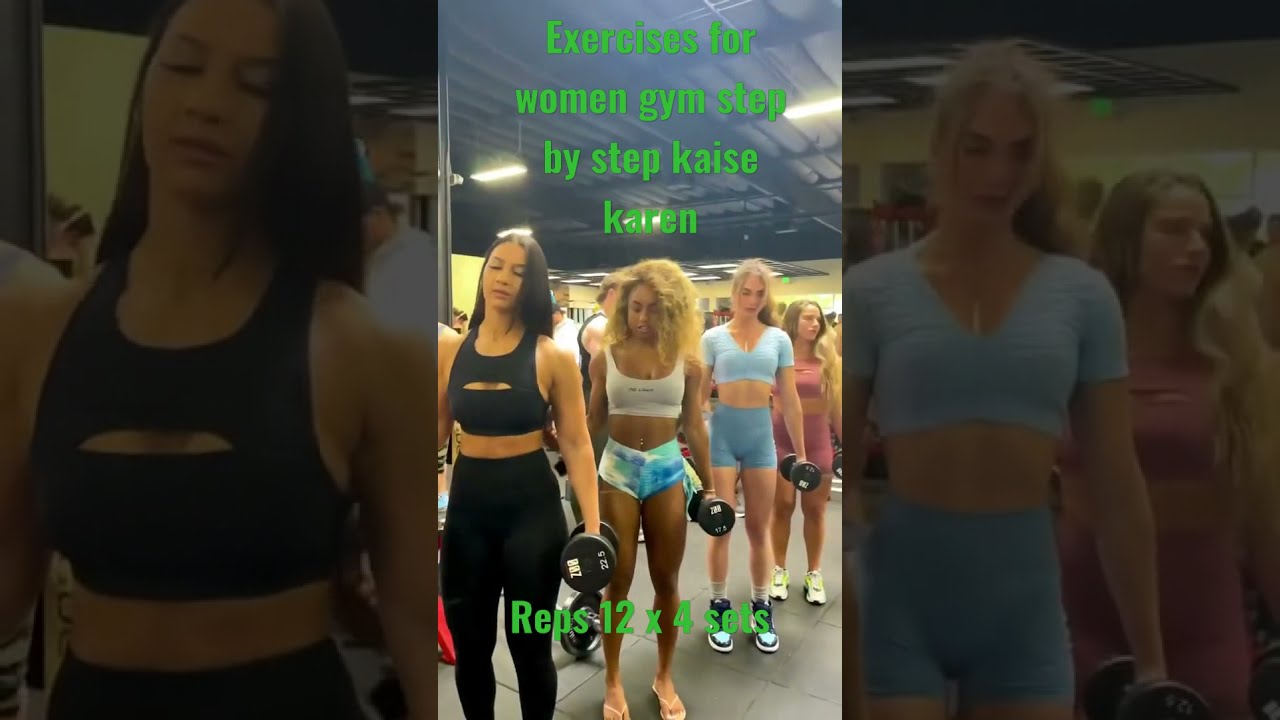The image showcases a line of women standing inside a gym, each holding round black weights in their left hands. They are dressed in athletic wear, ranging from black tank tops and leggings to crop tops and shorts of various colors. The front-most woman, characterized by her long dark hair, is dressed in a black sports bra and leggings. Behind her, another woman with frizzy blonde hair is wearing a white crop top and tie-dye blue shorts. Further back, a woman with long blonde hair is clad in a light blue crop top and matching biker shorts, followed by another blonde woman in a pink sports bra and pink cycling shorts. The background features a faded-out version of the same scene, with a closer focus on the woman in the black tank top. Text overlays the image, reading "Exercises for Women Gym Step-by-Step Case Karen" in green font, with "reps 12 by 4 sets" at the bottom. A wide, fuzzy border, created from close-up sections of the main image, frames the scene on both sides.